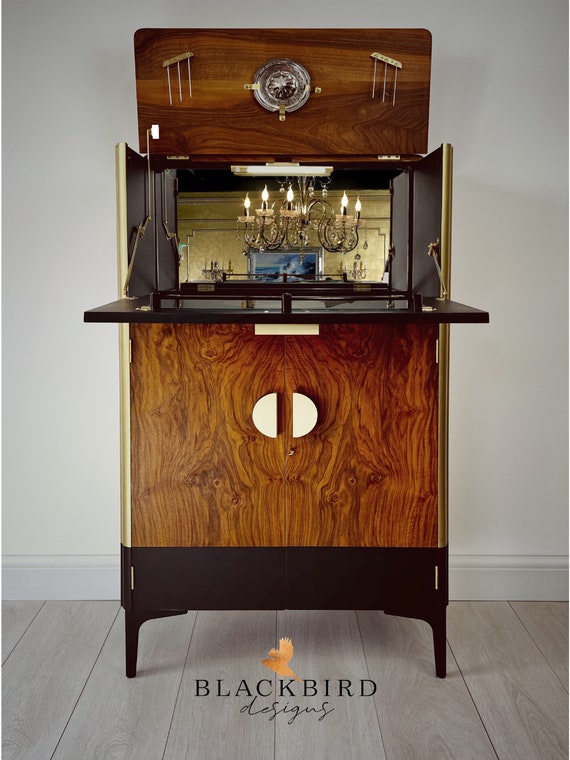The image captures a detailed close-up of a vintage cocktail cabinet made primarily of wood, positioned against a white wall with rustic, light gray wooden plank flooring. The floor is complemented with white molding along the wall bottom. The cabinet itself features a black base supported by thin black legs, and the bottom center displays the logo "Blackbird Designs" in black letters—the word "Blackbird" is capitalized in a bold font, with "Designs" in a script font, accompanied by a gold-colored bird flying above.

The lower section of the cabinet includes two large doors adorned with half-moon-shaped gold handles, providing a secure closure. Above this section is a black shelf, leading to two more upper doors that are currently open. Inside, the backing appears to be mirrored, reflecting a chandelier situated behind the photographer. The open upper section reveals what resembles a miniature living room, complete with a gold wall, a painting, and a small chandelier, giving an impression of an intricate, dollhouse-like interior. At the very top, a hinged wooden piece, designed to swing down and cover the mirror, is currently raised. The photograph is well-lit with natural lighting, highlighting the detailed craftsmanship of the cabinet in a bright and clear setting.